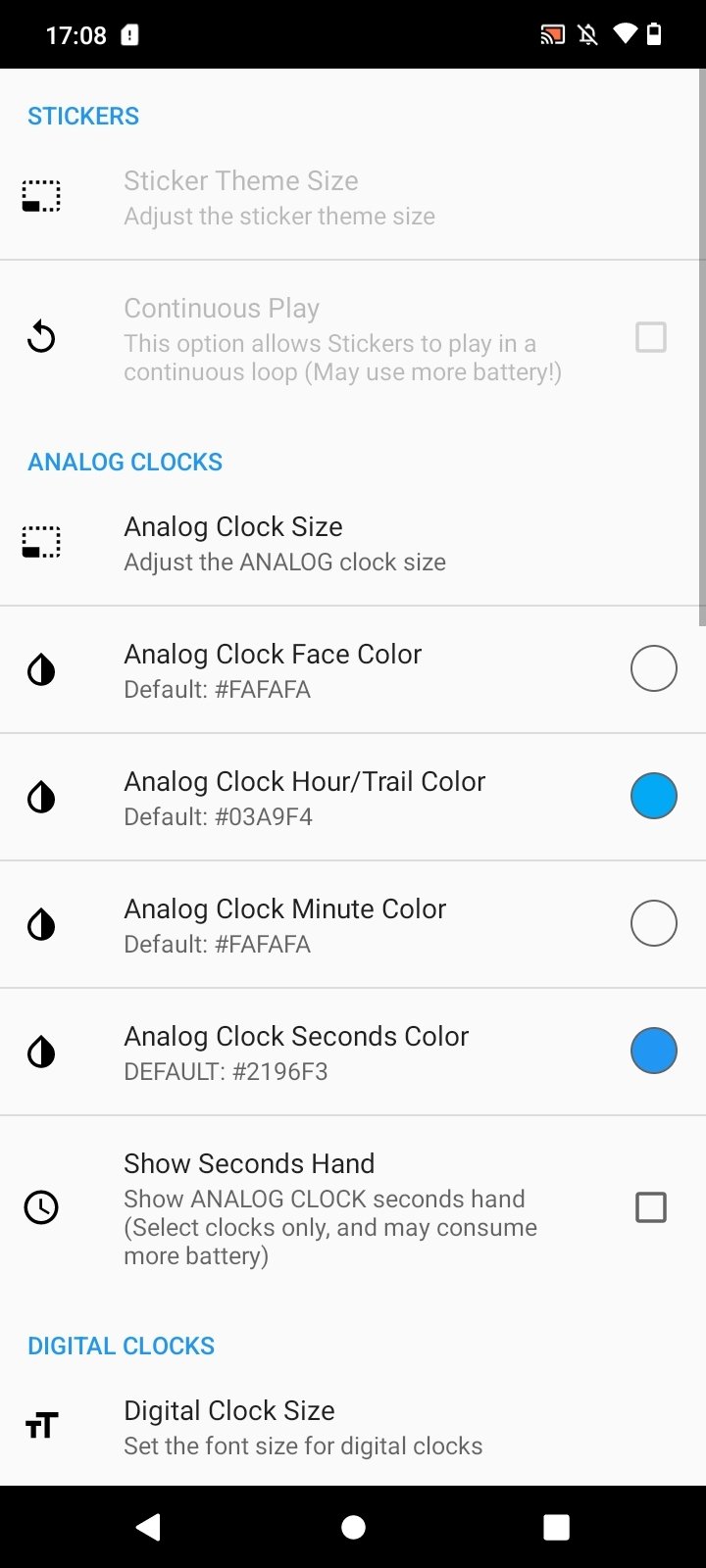**Caption:**

The screenshot, taken from a mobile device, displays the time at 17:08 in the top left corner. The top right corner showcases various status icons: a half-full battery, Internet connectivity, notifications muted, and a possible screen share icon indicating either an active or inactive status. The main part of the screen delves into settings for clocks. The top of the list includes options such as "Stickers," "Sticker Theme Size," and "Continuous Play." Below this, there is a section titled "Analog Clocks" with the following settings: "Analog Clock Size," and four different analog clock customization options: "Clock Face Color," "Clock Hour Trail Color," "Analog Clock Minute Color," and "Analog Clock Second Color." Notably, blue dots next to the "Clock Hour Trail Color" and "Analog Clock Second Color" suggest these options are selected or active. There is also an unchecked "Show Second Hand" option located here. Below these settings, a section labeled "Digital Clocks" is mentioned but not visible in the screenshot.